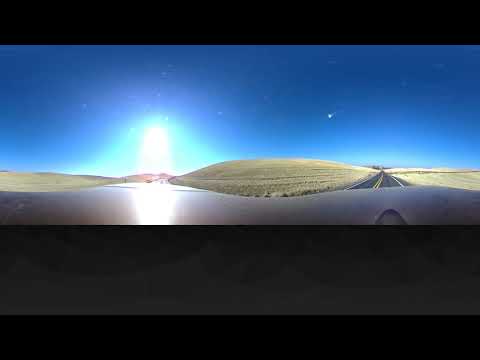The image is an expansive outdoor scene captured in a 360-degree panoramic shot from a vehicle on an empty road. The road runs along the right-hand side of the image, featuring two yellow lines down the center and white lines on the edges. It stretches into the distance, framed by rolling hills covered in green grass and some dry, brown patches. Towards the left, the sun is visible, casting a bright white light with a sea-green hue emanating from it, giving a reflective glow on the glossy black roof of the vehicle. The sky is a vivid blue, dotted with tiny white stars. A gentle grassy slope rises in the center of the image, adding to the serene landscape. The entire image is bordered by black rectangular strips at the top and bottom, with a gray strip above the bottom border, creating a layered framed effect.